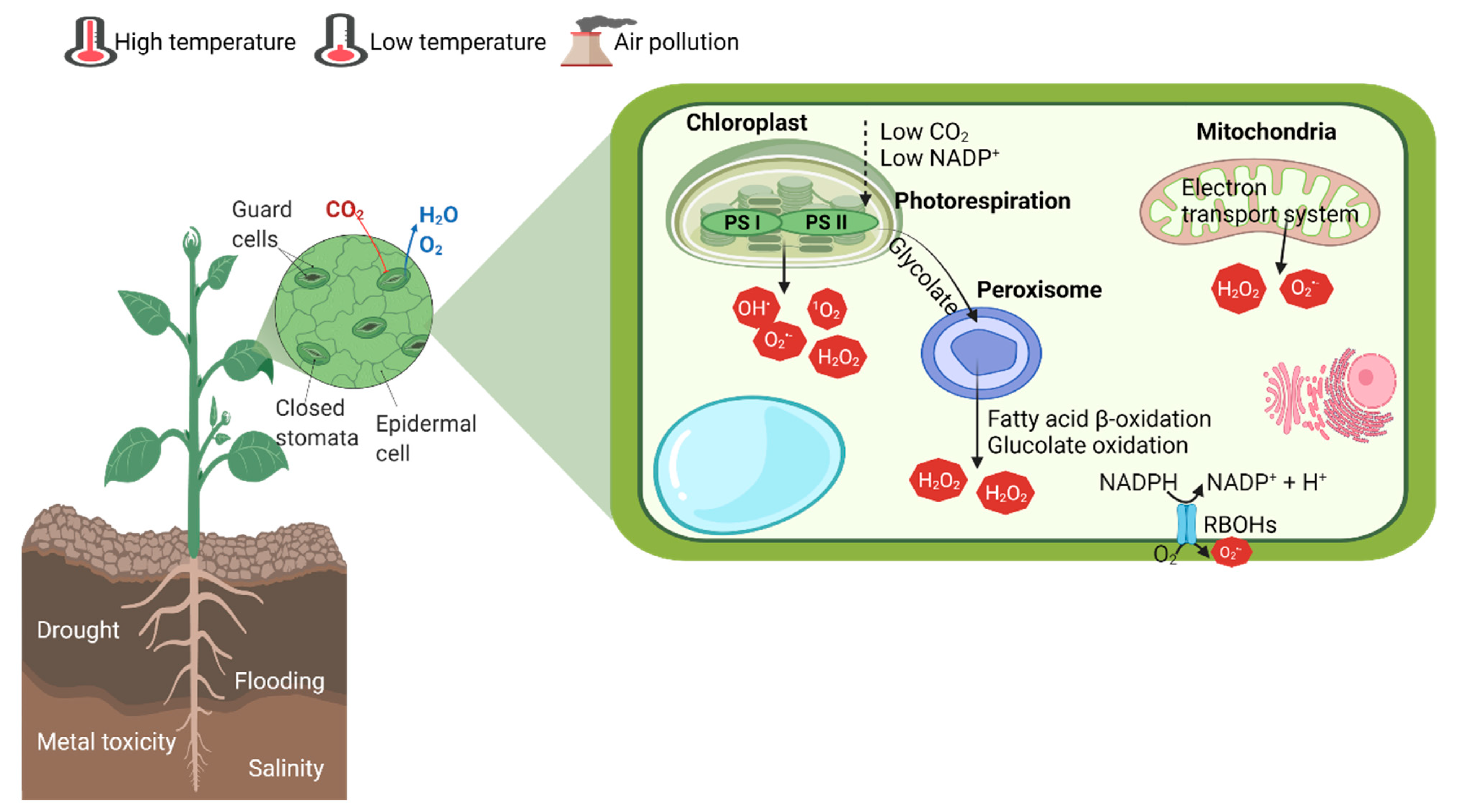This image is a comprehensive scientific diagram, potentially seen in a science book, journal, or magazine, illustrating various plant-related processes and environmental factors. 

In the upper left corner, there are symbols indicating high and low temperatures, represented by a pair of glass thermometers, and air pollution, depicted by a small building emitting smoke. On the left-hand side, the diagram features a cross-section of soil, showing two distinct layers: the upper layer is dark brown and crumbly, and the lower layer is light brown. Embedded in the soil are roots extending from a green plant. Labels indicate environmental stressors: "drought" and "flooding" are marked near the surface, while "metal toxicity" and "salinity" are indicated deeper down.

Zooming in on a leaf of the plant, the diagram highlights key components and processes within the plant's cells. Terms such as "guard cells," "CO2," "H2O," "O2," "closed stomata," and "epidermal cell" are annotated around the leaf structure. Further zooming in provides detailed labels of cellular components like "chloroplast," "fatty acid B oxidation," "glycolate oxidation," "mitochondria," "electron transport system," and various chemical symbols and scientific terms related to plant physiology.

Overall, this diagram intricately depicts the interactions between environmental conditions and internal plant processes, highlighting both macro and microscopic details.